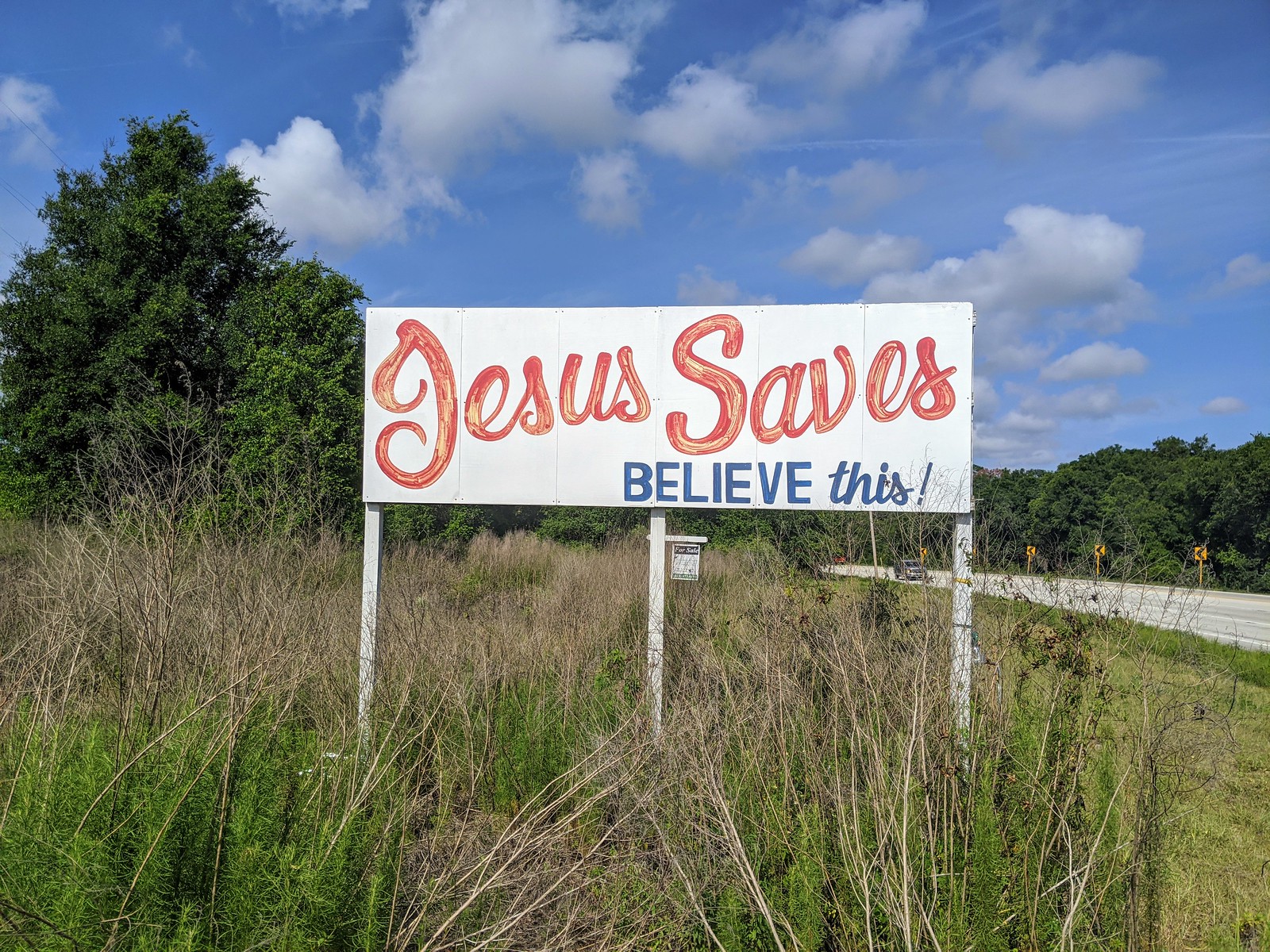This image depicts a roadside scene under a bright, deep blue sky adorned with a few white clouds. A prominent white sign, standing on three white posts, displays a religious message: "Jesus Saves" in red cursive font followed by "Believe This" in blue regular font. The sign is situated in the middle of an overgrown field consisting of green and brown plants. Nearby, a lush, leafy green tree stands behind the sign, while additional trees line the far right side of the paved road. The road, situated in the right-hand corner of the image, is light gray concrete adorned with yellow curve warning signs and features a single car traveling along it. The scene captures a quiet, rural atmosphere with a spiritual reminder prominently displayed amidst nature.